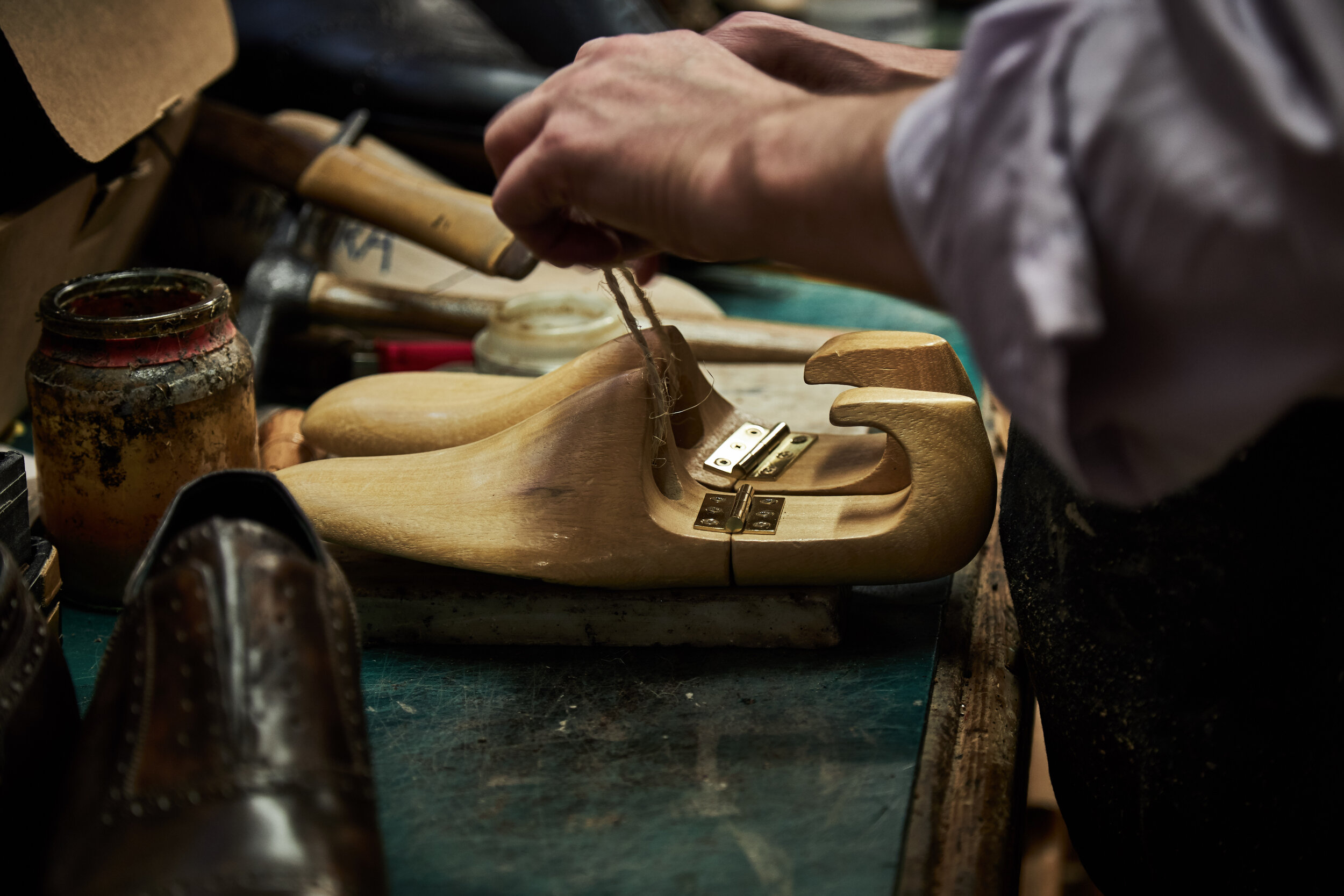In this detailed photograph, a shoemaker is meticulously at work, partially seen with his rolled-up long-sleeves exposing his wrists as he leans over a green table. His hands grasp rope-style laces connected to a pair of intricately crafted wooden shoe frames, each featuring a brass latch in the middle. These wooden pieces, smooth and light brown, are designed to resemble the ends and backs of shoes. A hollow space inside and a string protruding from them hint at the intricate craftsmanship involved. Scattered on the table is a partially visible worn leather shoe with no laces, alongside jars possibly containing shoe polish, including a well-worn, splattered jar in yellow, red, and black. In the left corner of the frame, there's a shiny brown leather shoe, hinting at the shoemaker’s dedication to his craft. Tools arrayed behind the man complete the busy, industrious scene.